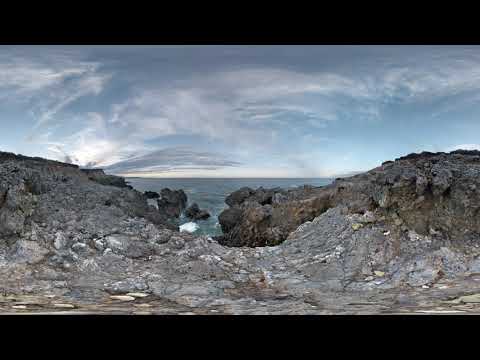The photograph captures a rugged coastal scene, framed by black bars at the top and bottom that give the image a letterbox effect. The terrain is characterized by brown and gray rocky hills on the left and right, which converge into a central gap, revealing a teal to blue-gray waterway that seamlessly extends into an open ocean. The rocky surface, littered with fine lines and cracks, varies in color—darkening further from the viewer and lightening up close. The stones look inhospitable and unstable. Overhead, a partly cloudy sky, filled with swirling white and gray clouds, stretches across a pale blue canvas. The lack of bright daylight suggests the photo was taken during a subdued day, possibly approaching evening. The pixelation and slight warping hint that the image might have been taken with an older digital camera.